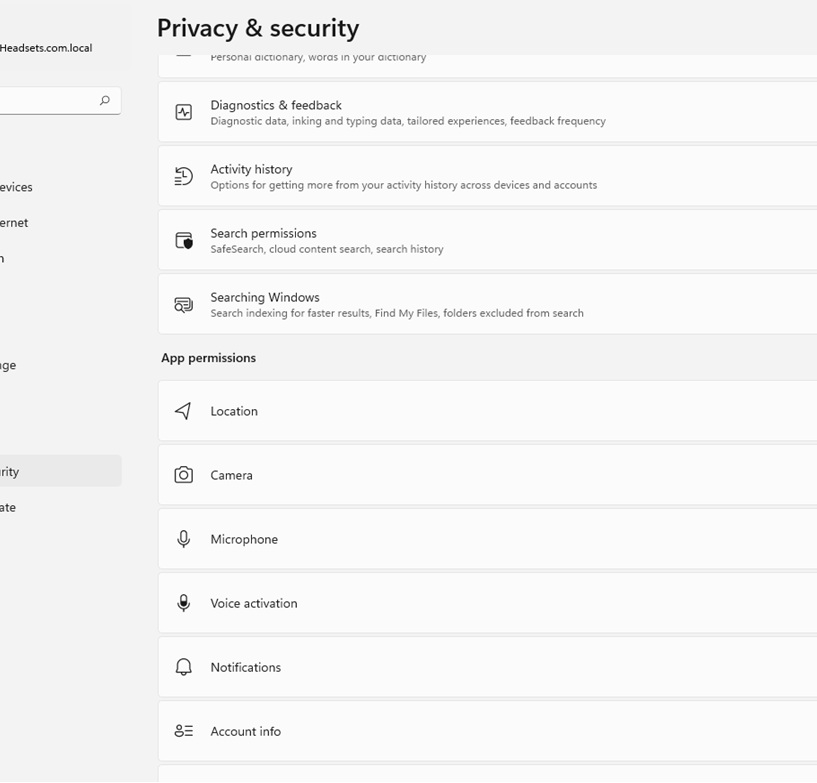A partially visible screenshot captures a section of a device's Settings menu, focusing primarily on the "Privacy and Security" category. The left side of the image includes a truncated, partially obscured sidebar with a search bar positioned at the top left. The right side of the image showcases various settings options under the "Privacy and Security" heading, slightly scrolled down, starting with "Diagnostics and Feedback." Visible options include "Diagnostic Data," "Inking and Typing Data," "Tailored Experiences," and "Feedback Frequency."

Further down, the "Activity History" section presents options to manage activity history across devices and accounts. Below it lies the "Search Permissions" set, encompassing settings such as "Safe Search," "Cloud Content Search," "Search History," and "Searching Windows," along with "Search Indexing for Fast Results," "Find My Files," and "Folders Excluded from Search."

The last readable section is "App Permissions," listing permissions for "Location," "Camera," "Microphone," "Voice Activation," "Notifications," and "Account Info." The image provides a glimpse into the detailed configuration options available for ensuring privacy and security on the device.